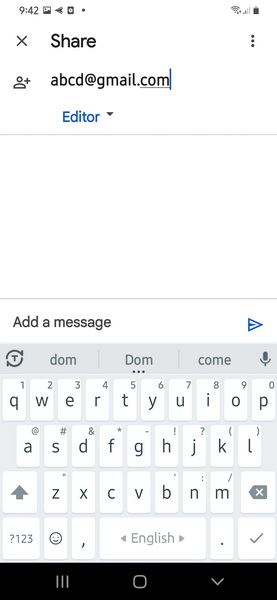The image displays a smartphone screen with a fully charged battery and a strong connection signal, indicating it is 9:42 AM. At the top of the screen, there is a prominent "Share" button in bold black letters, alongside an "X" icon on the left and three vertically aligned dots on the right. Below these icons, the email address "abcd@gmail.com" is visible. 

Further down, there is an icon of a person with a plus sign next to it, and the word "Editor" in blue lettering, accompanied by a dropdown arrow. Following this, a blank white space occupies the middle portion of the screen.

Below the white space, there is a section labeled "Add message," featuring a text input field. Above the keyboard, text suggestions like "Dom" (with a capital D) and "come" are displayed. The on-screen keyboard includes the standard alphabet keys, with "English" indicated in the middle. Additional keys include an emoji button (smiley face), a "1 2 3" button with a question mark, and an arrow. There's also a microphone icon indicating voice input capability. This setup shows how one might begin typing a message just as they would when texting on any smartphone.